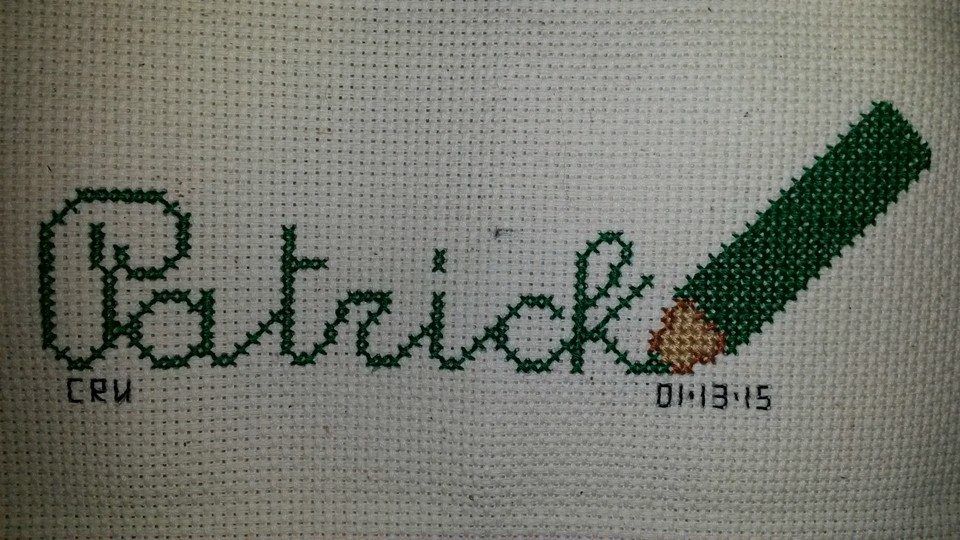The image is a landscape-oriented color photograph showcasing a cross-stitched design. The background is white cross-stitch fabric. The main focus is the name "Patrick," which is elegantly stitched in a script font with dark green thread, spanning from the left side to about three-quarters across the fabric. To the right of the name and seamlessly integrated, a dark green, wide colored pencil with a beige tapered tip appears to be drawing the name, specifically pointing to the descender of the letter "K". Below the pencil, the date "01-13-15," presumably marking the creation date of the piece, is stitched in the same dark green thread. The initials "CRW" are carefully stitched in all caps beneath the "P" in "Patrick" in the bottom-left corner. The overall style of the piece reflects photographic representationalism, capturing the detailed realism of the handcrafted item.